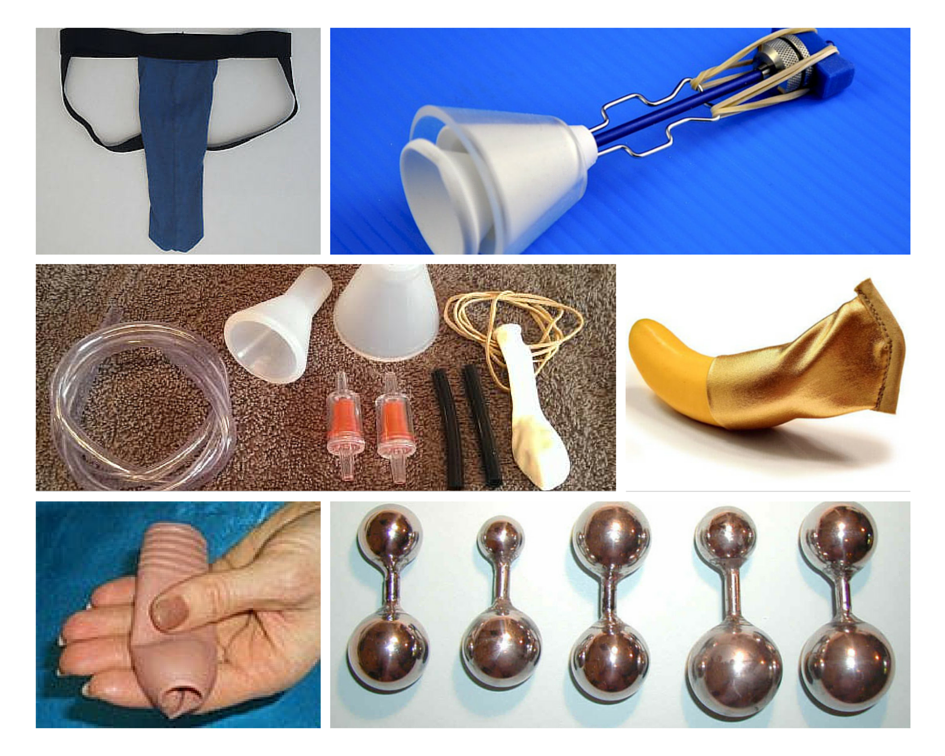This collage features six distinct images, each showcasing a unique object. In the top left, there is a black jockstrap with a dark blue fabric in the middle, resembling a phallic shape. To its right on a blue backdrop is a kitchen utensil with a white top and a metal handle, featuring a blue bar held by rubber bands and a suction cup at the bottom. Centered in the collage, against a rose-colored carpet, are various miscellaneous items: plastic tubing akin to nebulizer attachments, two humidifier parts, a white balloon, a piece of small twine, two black stick-like objects, and a funnel-shaped item. To the immediate right of this central image is an image of a yellow banana partially covered by a piece of golden fabric, against a white background. The bottom left photograph displays a woman's hand, showcasing camel-colored fingernail polish, holding a skin-toned phallic-shaped object, with a blue background. The bottom right image shows several metallic barbells, possibly used for Kegel exercises, set against a light blue background.